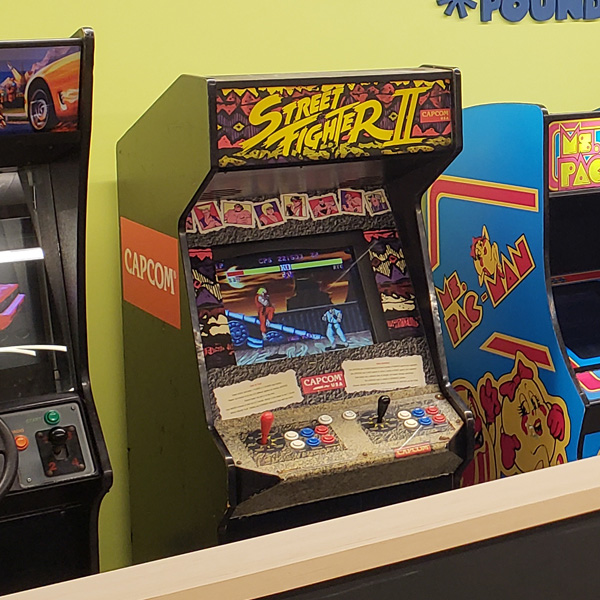The image showcases a nostalgic scene of classic arcade video games. Prominently featured is a Street Fighter II arcade machine by Capcom, recognized by its black exterior and distinct branding. The cabinet displays the game's title at the top, and surrounding the screen are illustrations of characters in combat. The game interface reveals two characters in mid-battle with health bars displayed above. The control panel beneath the screen is equipped with a variety of buttons in white, blue, and red, along with joysticks for two-player interaction.

Flanking this central arcade machine, to the left, a portion of another black arcade game is visible, though its name is unreadable. It features a noticeable green and red button. On the right side of the image stands a third arcade cabinet, shorter and painted in blue with bold red lettering declaring it as Ms. Pac-Man. This machine is adorned with an image of Ms. Pac-Man herself and bears additional branding on its front, though only partially visible. The scene is framed by a dark gray wall with a white ledge in the foreground, adding depth to this nostalgic glimpse into vintage gaming.